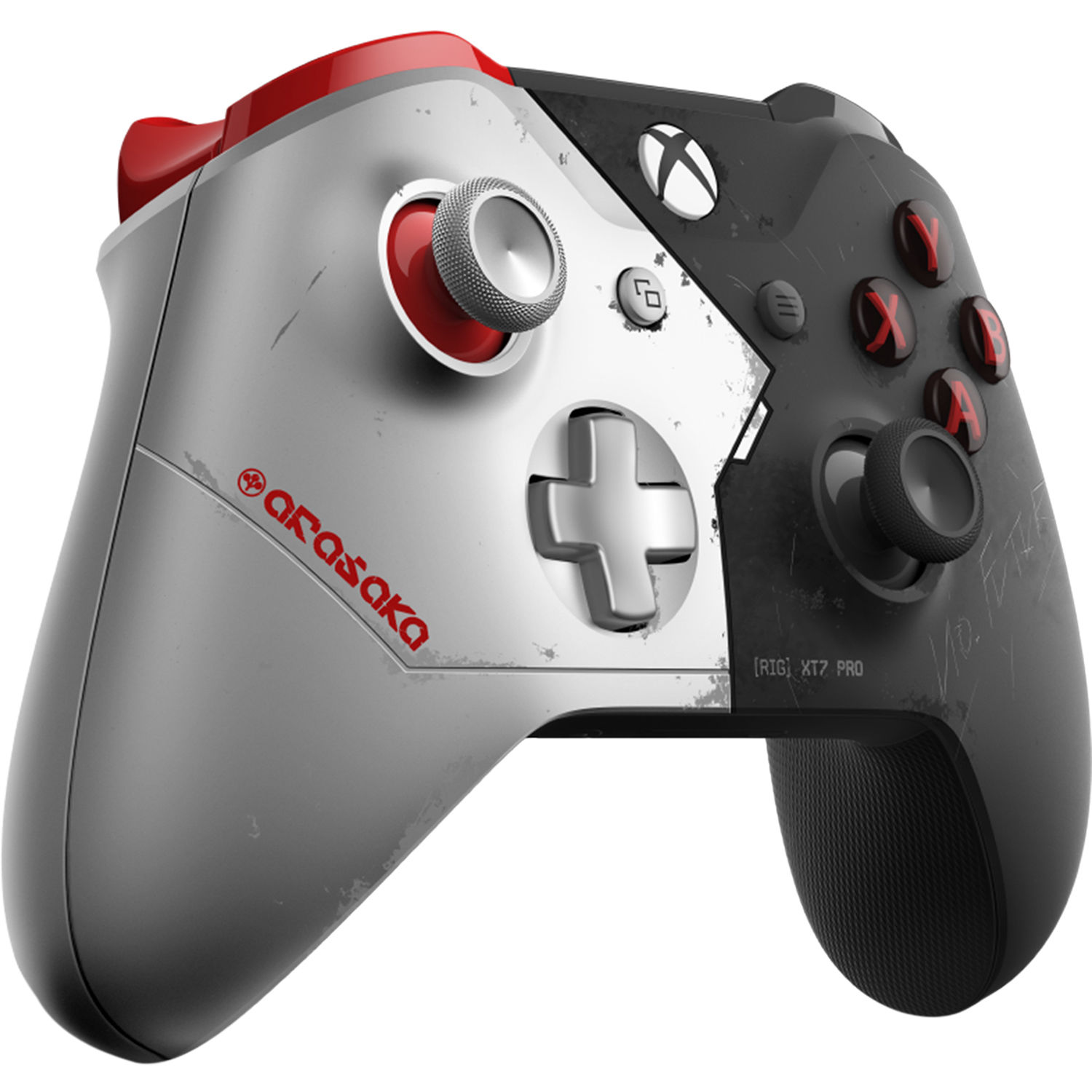This detailed photograph showcases a well-used video game controller, distinctly attributed to the Arasaka brand. The controller features a unique dual-tone design, with the left side being gray (silver) and the right side black. Prominently in the center, there is a cross directional button enabling navigation in north, south, east, and west directions. Spread across the black portion are four black buttons inscribed with red letters: X, Y, B, and A. Additionally, there is a large control knob likely used for navigation. An array of other buttons includes one with three horizontal lines and another white button marked with a red 'X'. A notable detail is the presence of silver text on the black side, reading "RIG XT7 Pro". Red accents are visible around the directional control knob, complementing the red text that spells "ARASAKA". The device also features an "Xbox" symbol at the top, cementing its identity as a gaming handheld device. The word "Vioforte" is written on it, further adding to its detailed aesthetic and functionality.